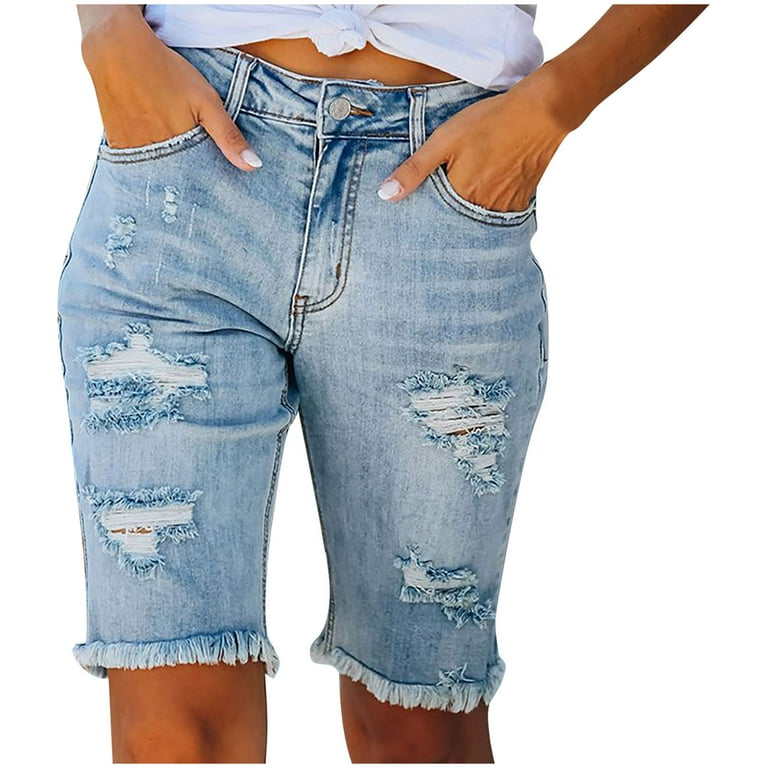In this stock photo, a tan-skinned woman is depicted wearing light blue, distressed jean shorts that end just above the knee with frayed, unhemmed edges. The frayed edges are about an inch long, giving the shorts a rugged appearance. The shorts showcase multiple rips, including two prominent ones on the left and right sides. The woman has her hands tucked into the shorts' pockets, revealing her well-manicured French tip nails. She is also wearing a white crop top that's tied in a knot above her navel, exposing a small portion of her midriff. The backdrop of the image is a blank white background, emphasizing the focus on the woman’s attire and her tan complexion.